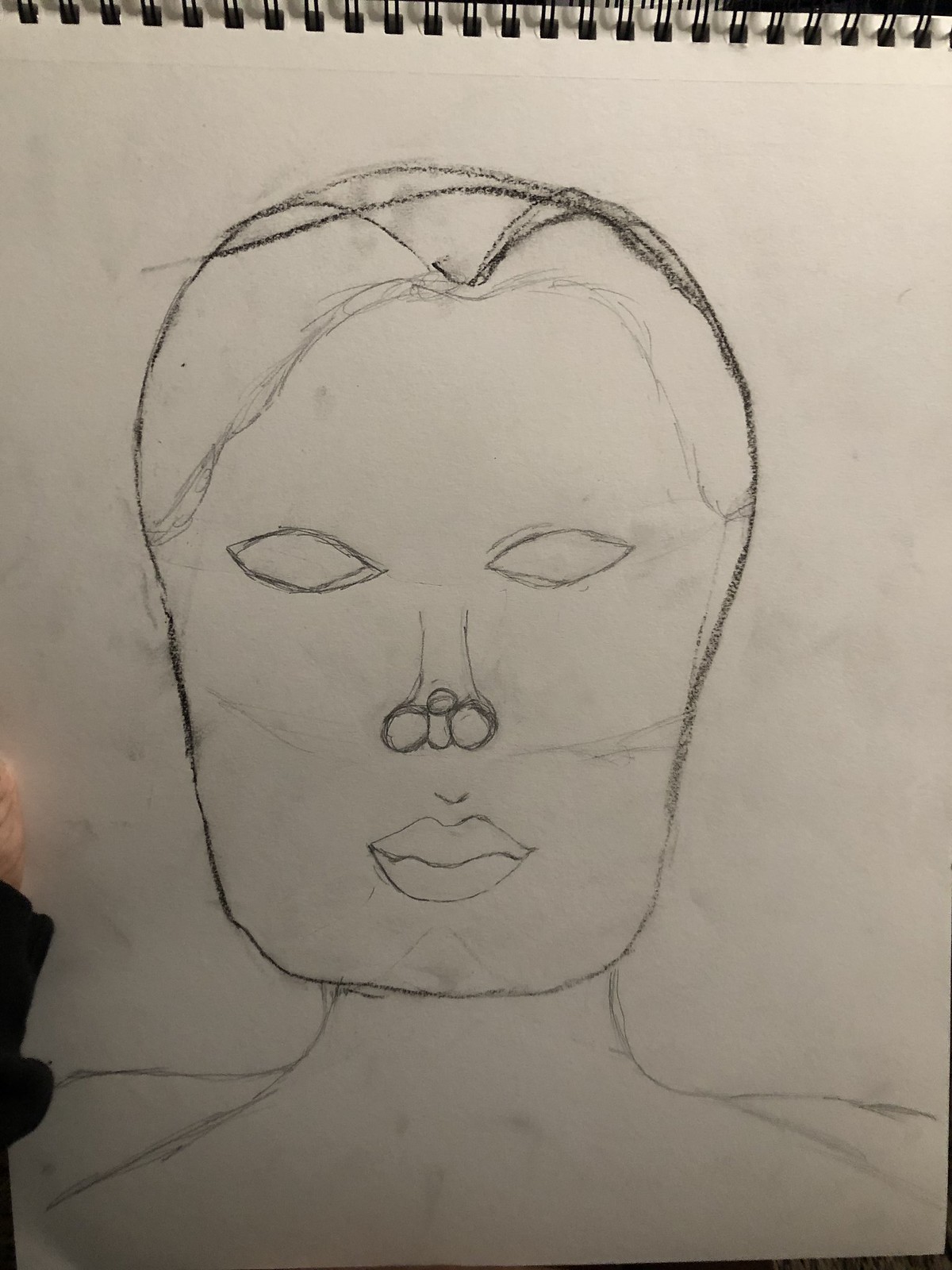The image presents a well-lit photograph of a spiral-bound sketchbook held by an individual whose plaid shirt sleeve is visible in the left corner of the frame. The sketch, drawn on a blank page, features an attempt at creating a human face, suggestive of someone learning or practicing drawing techniques. The face itself is quite rudimentary, with characteristically oval eyes and a pair of semi-realistic lips. The head is uniquely shaped, leaning towards an elongated oval. Various circles indicate the nostrils, contributing to the odd appearance of the nose. Additionally, preliminary lines depict hair, framing the incomplete face. The figure’s shoulders are drawn in two differing styles—broad and slightly angled inward—revealing the artist’s indecision on the body’s proportion. The ambiguity of the gender is further accentuated by the absence of ears and the lack of defining features.